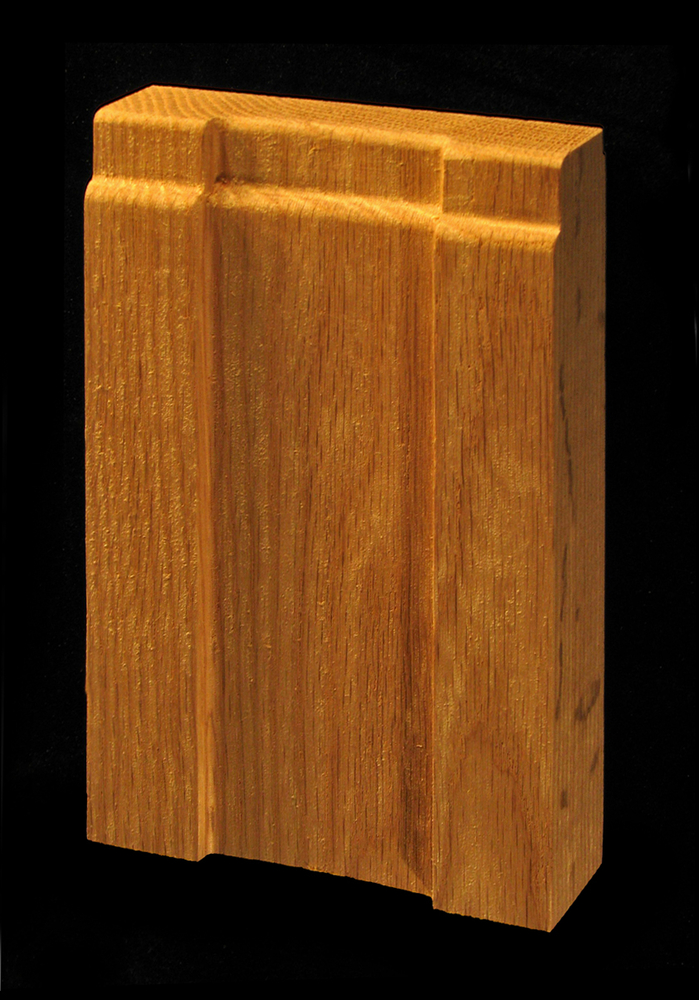This detailed photograph showcases a unique block of wood against a black background. The block is slightly taller than it is wide, approximately four inches in width and an inch in depth. Carved from what appears to be oak, the wood displays an array of grain patterns—on the left side, the grains are close-knit and straight, while on the right side, they are more curvaceous with blonde and lighter streaks, suggesting it might have been stained. The wood features an intricate design with two raised ends and a step-like middle, creating a central groove that is about two inches wide, flanked by half-inch edges. Additionally, there is a smaller notch on the top, hinting at a functional purpose, possibly as a component in a larger construction, such as a bed slat. The craftsmanship is evident with one end appearing to be cut and the other sanded. This nuanced design implies that it might fit snugly into another piece, potentially designed to be hammered in for assembly.